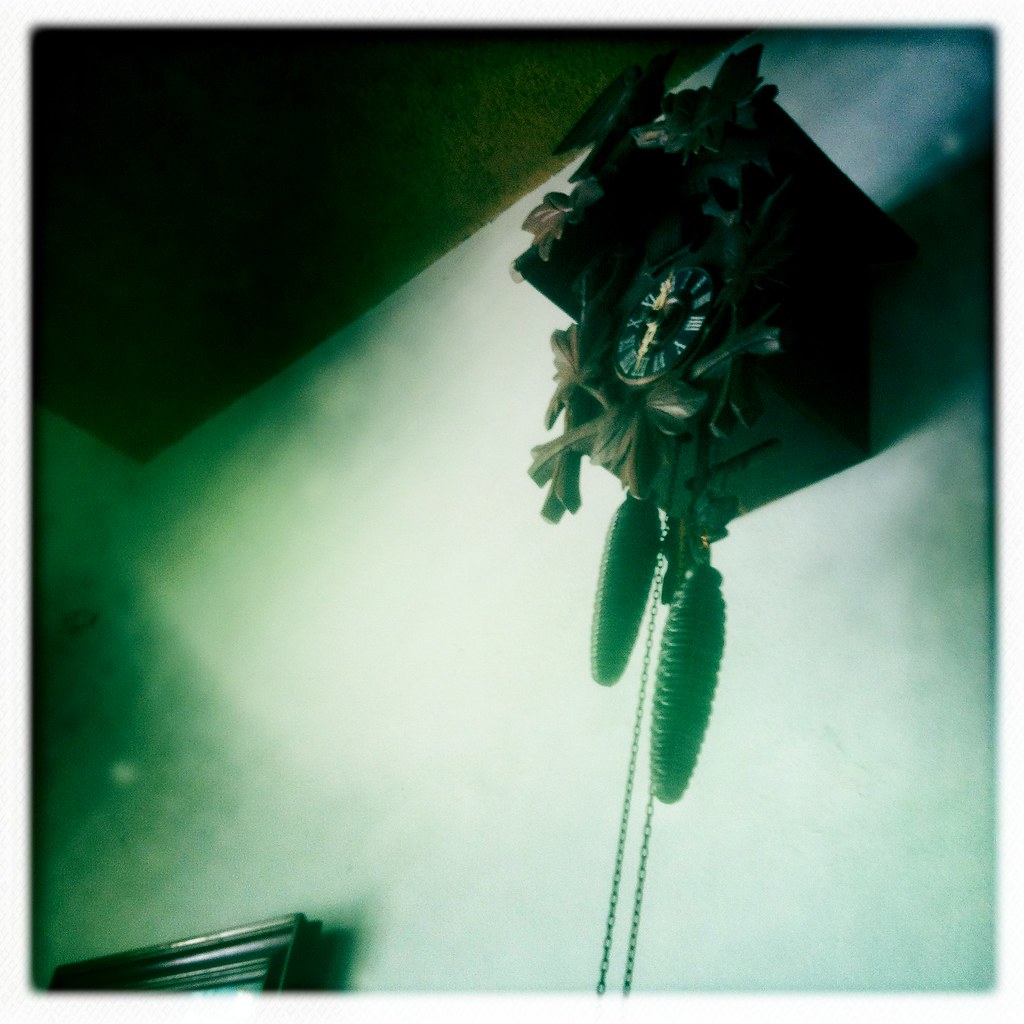A high-angle photograph showcases an ornate cuckoo clock mounted high on a wall, near the ceiling. The image is rendered in a grainy, aged style with a green and blue tint, suggesting the utilization of a vintage filter. The clock is framed by an intricate border featuring carved leaves, and the chimes hanging below resemble pine cones. At the pinnacle of the clock, a delicately crafted bird sits, adding to the clock's old-world charm. The color filter gives the scene a surreal, nostalgic ambiance.